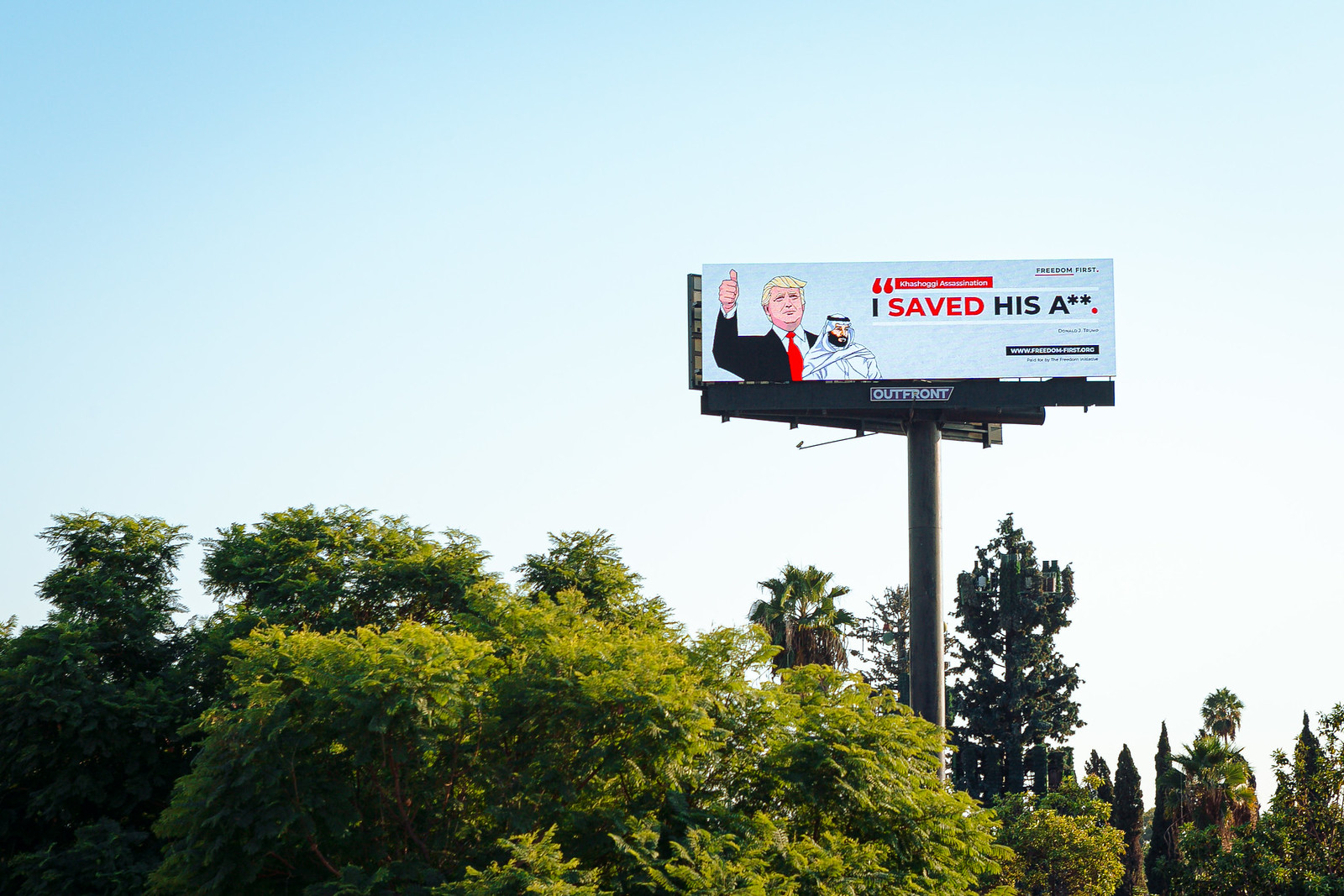In this exterior image taken on a bright, clear day, a black-framed billboard dominates the right-center portion of the scene. The billboard is mounted on a dark gray, cylindrical metal pole that rises above a mix of tall trees with light and dark green leaves. The sky forms a gradient from light blue at the top to white, creating a crisp backdrop. The billboard itself, a narrow horizontal rectangle with a light blue background, features an animated depiction of former President Donald Trump on the left, dressed in a black suit, red tie, and sporting his signature blonde hair. Trump is shown with his right thumb raised. To the right of Trump stands a smaller figure of an Arab man in a white robe. The text on the billboard reads, "I saved his A**," with "saved" in red and the rest of the phrase in black, enclosed in quotation marks. The bright lighting in the image is coming from the right side, emphasizing the billboard’s details.